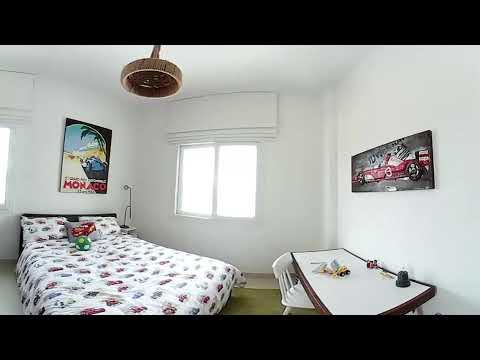The image depicts a child's bedroom adorned with a car theme. Situated indoors, the room has a white wall in the background featuring a window centrally located. On the right-hand side, a painting of a red race car with a gray background is mounted on the wall. Below this painting is a white table with a brown border, displaying several small toys, and paired with a white chair.

Across from the table is a neatly made full-size bed positioned on the left-hand side of the room. The bed is covered with a comforter decorated in white, red, and blue race car designs, accompanied by a set of pillows including a green and white eggshell pillow, two additional white pillows, and a gray pillow with a red image.

Above the bed hangs another car-themed poster, emblazoned with the word "Monaco" in red, featuring a car driving scene. The room has a wicker ceiling light installed centrally, contributing to its cozy aesthetic. The overall decor and details suggest that the room belongs to a young boy with an interest in race cars.